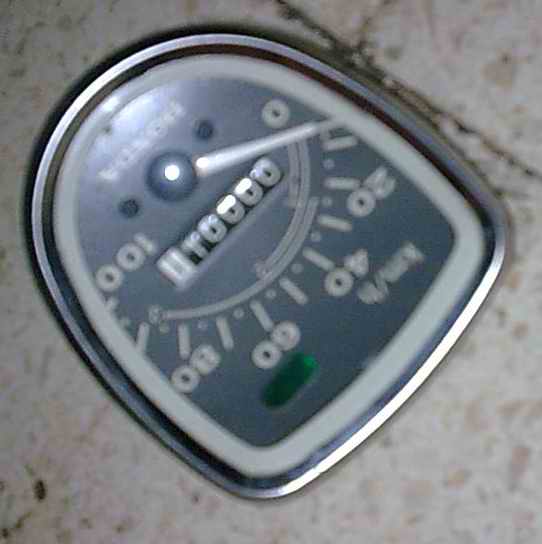This is an inverted photograph of a motorcycle speedometer, situated on a tile or marble floor. The image is angled from the top-left to the bottom-right corner, with the upper section oriented towards the right. The speedometer resembles an inverted 'U' shape with a white-bordered inner section. The dial face is gray with white text, displaying speed in kilometers per hour, and the total mileage reads 1.1. At the bottom, there's a Honda insignia, and a light silver dial indicator shows the speed. This component appears to be a spare part for replacing the speedometer on a Honda motorcycle, depending on the model.